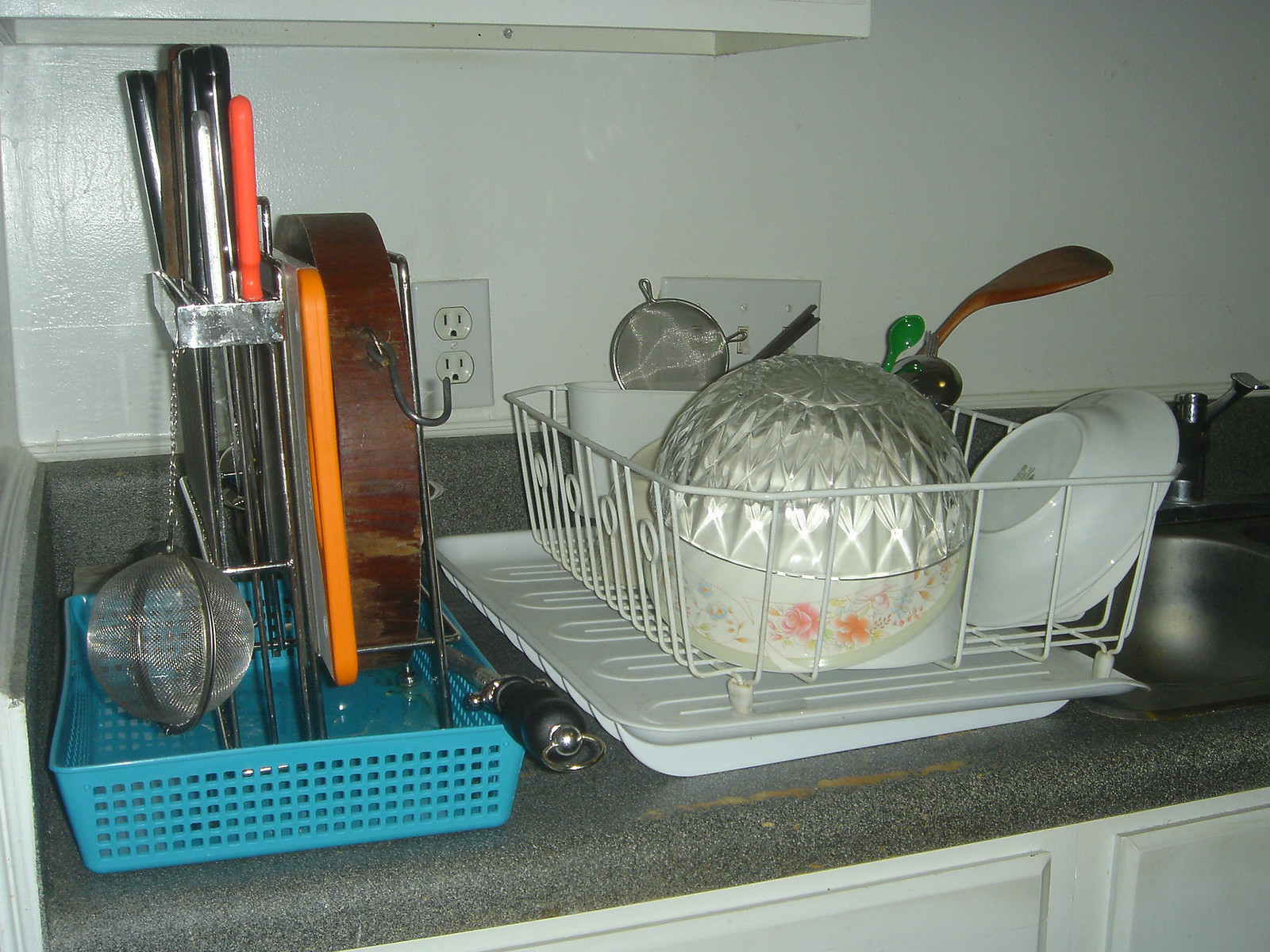The photograph depicts a tidy kitchen setting, focusing closely on a stainless steel sink with an adjoining faucet. The walls of the kitchen are painted white, creating a clean and bright atmosphere, while the gray laminate countertop provides a sleek and modern contrast against the white cabinets below.

To the left of the sink, a white wire dish rack holds an assortment of kitchen items. Among these, a clear glass bowl with a crystal-like design catches the light, sharing space with a white CorningWare bowl adorned with pink and orange floral patterns, complemented by blue accents. A neighboring white pasta dish bowl completes the ceramic collection. Positioned prominently in the dish rack are also various utensils: a wooden spatula, a green plastic spoon, and a stainless steel mesh sieve. 

Further to the left, a tall blue perforated bin serves as a kitchen utensil holder, from which a stainless steel tea strainer dangles. This bin accommodates several long knives and other varied kitchen tools, along with two mysterious items—one brown and one orange—that remain unidentified. 

In the background, a white wall-mounted light switch with three switches adds a functional element to the setting, while another white electrical outlet subtly blends into the white walls, ensuring the kitchen is equipped with necessary electrical amenities.